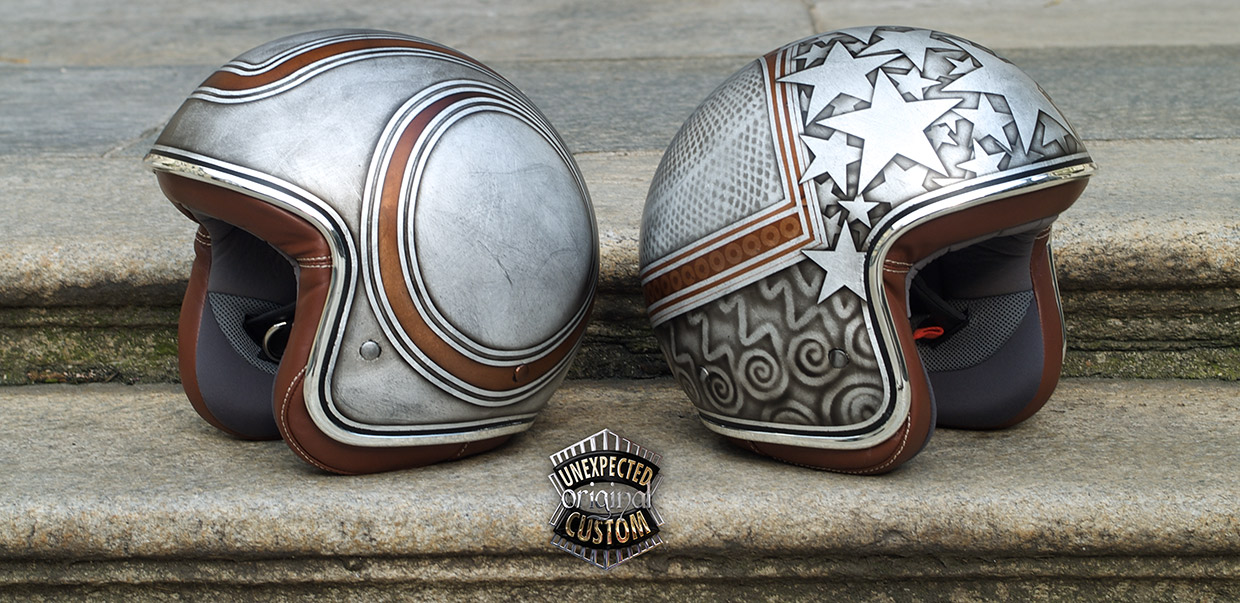In the image, two silver helmets with brown highlights are resting on worn, light gray concrete steps. The steps have mildewed and moldy edges, giving them a dark, weathered appearance. On the left, one helmet features a large brown circle on its side and has a dark gray inner lining. On the right, the other helmet is adorned with star outlines, a hammered diamond edge, and intricate squiggles at the bottom. Both helmets share a silver and brown color scheme. A logo positioned at the bottom center of the image reads "Unexpected Original Custom." In the background, another concrete step is visible, continuing the worn, gray aesthetic.